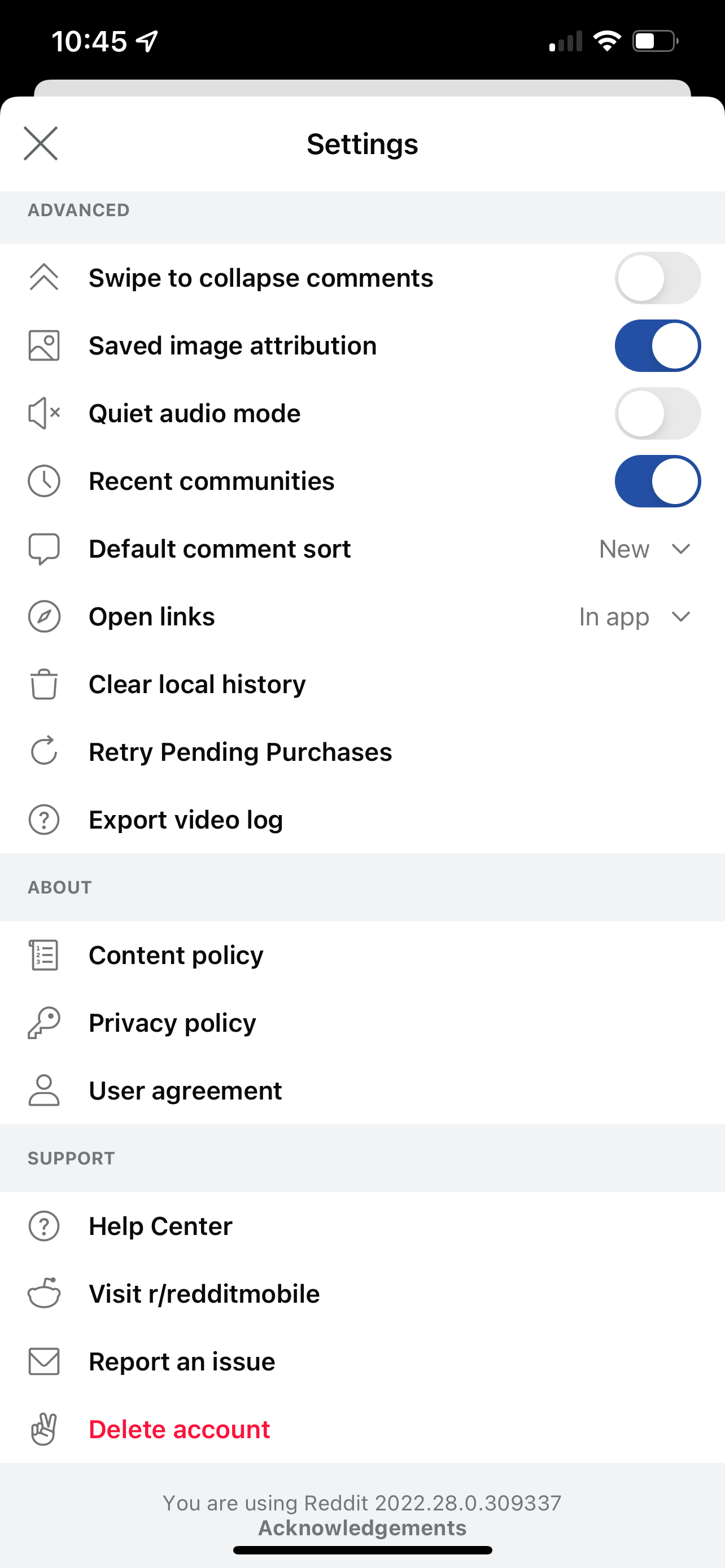The image depicts the settings menu of a Reddit mobile app on a smartphone, providing various customization and account management options. At the top, encased in a black bar, there is information about the time (10:45 on the left side), battery life (about half full), and weak signal strength (one bar) on the right. The background is predominantly white, contrasting with the detailed settings options.

The visible sections of the settings menu include:
1. **Advanced Settings**:
    - **Swipe to Collapse Comments**: Disabled.
    - **Save Images**: Enabled.
    - **Quiet Audio Mode**: Disabled.
    - **Recent Community**: Enabled; indicated by a blue slider button.
    - **Default Comment Sort**: Set to "New".
    - **Open Links**: Currently set to open within the app; changeable.
    - **Clear Local History**: Option available.
    - **Retrieve Pending Purchases**: Option available.
    - **Export Video Log**: Option available.

2. **Informational Sections**:
    - Gray box labels for:
        - **About**
        - **Content Policy**
        - **User Agreement**
    - Acknowledgments at the bottom of the screen.
    - Explicitly highlighted in red, the option to **Delete Account**.
    
3. **Additional Options**:
    - Gray box including options for:
        - **Help Center**
        - **Visit Reddit Mobile**
        - **Report an Issue**
        - **Delete Account** (highlighted in red)
    
   Finally, the bottom of the menu states, "You are using Reddit 2022," indicating the version of the application.

This organized and detailed caption provides a comprehensive description of the settings menu, emphasizing its functionalities and navigational elements.